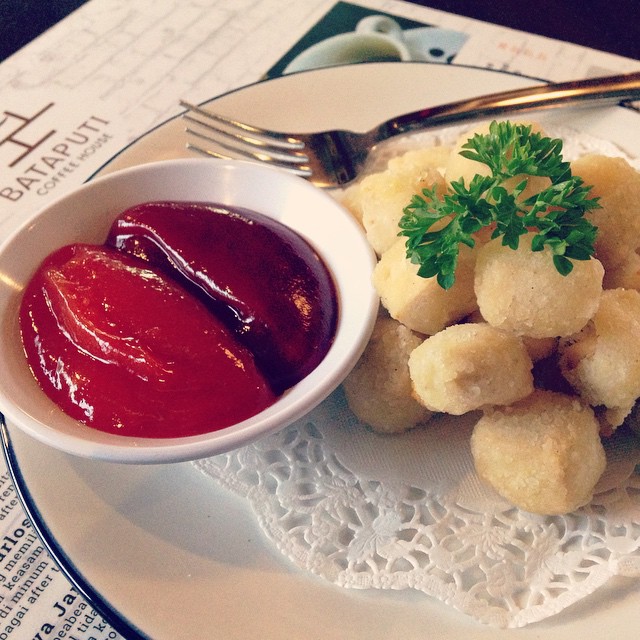This detailed close-up photograph showcases a plate of food ordered from Bataputi Coffee House, emphasizing the table setting and the dish. The white plate with a blue rim features a delicate white lace doily, upon which several small, round, fried cheese balls are arranged. These light yellow cheese balls are evenly breaded and garnished with a sprig of parsley, adding a touch of color. Beside them lies a small white ramekin with two distinct sauces: a bright red one resembling ketchup and a darker, glossy burgundy sauce, potentially a type of plum or barbecue sauce. A silver fork is set atop the plate, ready for use. The entire setting rests on a table adorned with a placemat and a visible menu displaying the name "Bataputi Coffee House." In the background, a faint image of a coffee cup subtly ties in with the café's theme.